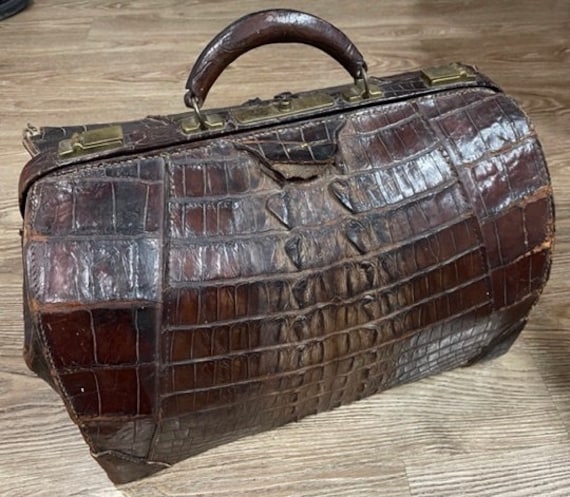This image features a single, vintage crocodile or alligator skin bag, possibly a doctor's bag, briefcase, or suitcase. The bag is predominantly brown with varying shades, including a lighter brown pattern in the middle, resembling a classic crocodile skin texture. It looks quite worn and slightly ripped, adding to its antique charm. The bag has bronze or brass clasps and decorations along the top, contributing to its aged appearance. An arched, darker brown handle extends straight up from the back. The bag, which appears to be about 10 inches to a foot across, is positioned on a floor with a grayish-beige wooden tone that features light to darker brown swirls.